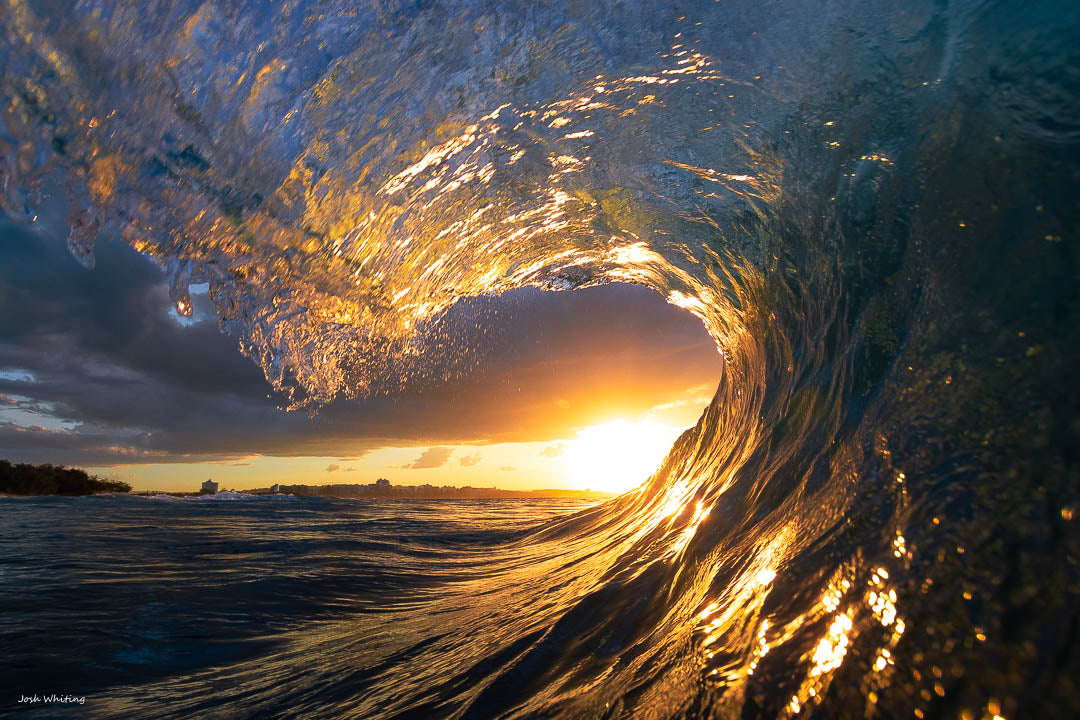This is a professional landscape photograph captured by Josh Whiting, as indicated by his small, white signature in the bottom left corner. The image presents a stunningly detailed view from inside the barrel of a massive, curving ocean wave. The wave's crystal-clear blue water contrasts deeply with the dark, textured sea below, which reflects the radiant light of an orange and yellow sunset on the horizon. The sunlight streams through the wave, casting golden streaks and intricate reflections along the inside of the barrel, creating a mesmerizing interplay of light and color. The top of the wave transitions to a pale blue with lighter gold highlights from the setting sun. Above, heavy dark clouds obscure part of the sky, yet patches of bright blue sky peek through, adding further depth and contrast. The scene is devoid of any human habitation, emphasizing the natural beauty and serene power of the ocean. The combination of technical precision and artistic composition makes this photograph both striking and relaxing, capturing a moment of pure, untamed nature.